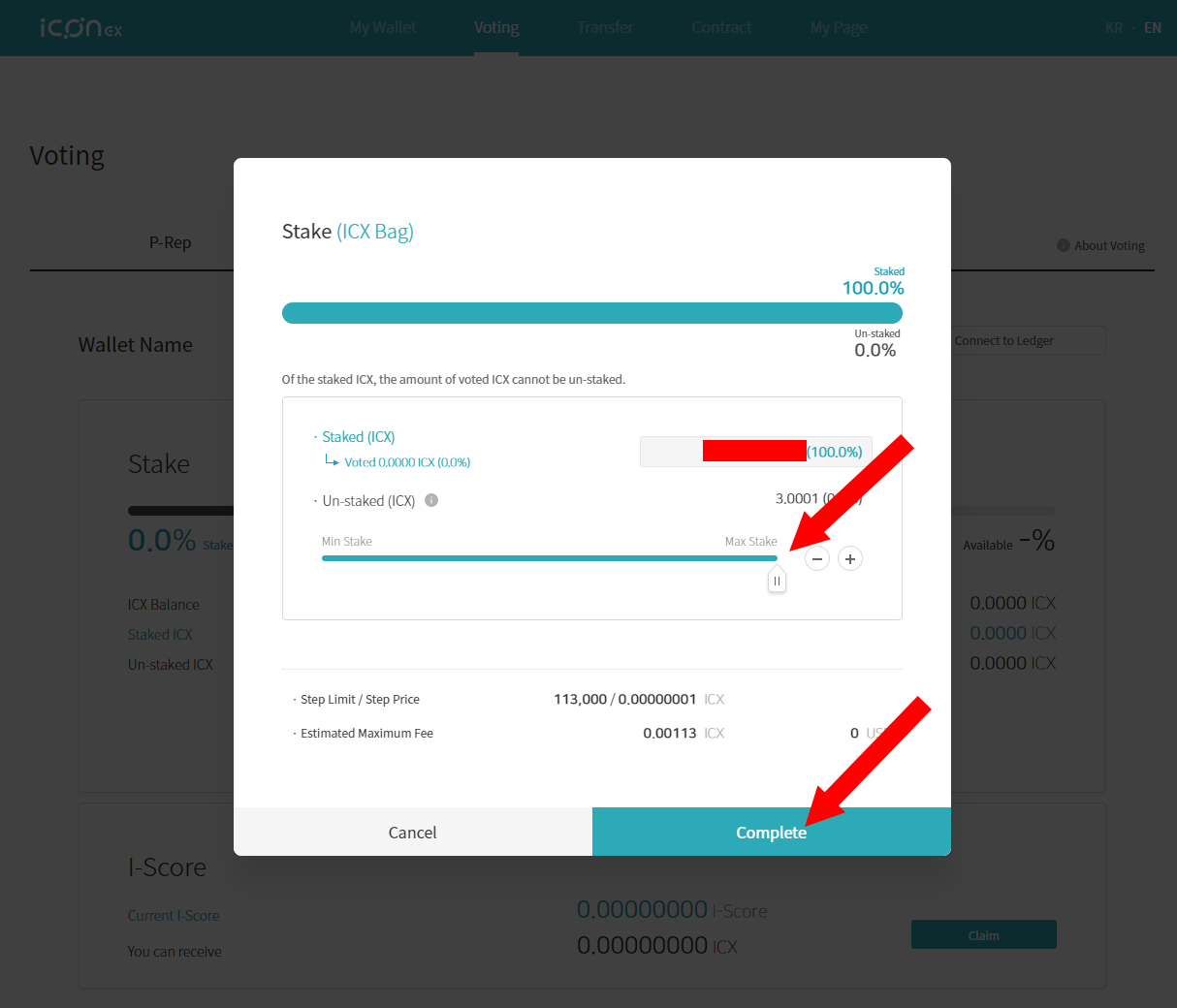The image depicts a webpage with the background grayed out, revealing a site named ICONX. The website's title, "ICON," is in large letters followed by "X" in smaller letters. Several tabs are visible in the background, with the "Voting" tab selected, showing the voting interface.

In the foreground, a pop-up window is prominently displayed, featuring a white background with green accents. At the top left of this window, the word "STAKE" is written, with "ICXBAG" in green within parentheses. Directly below this, a green progress bar, indicating 100% completion, stretches across, labeled "STAKE progress bar." 

Two arrows are visible on the pop-up. One points to a "MAXSTAKE" slider bar, which is set to its maximum position. The other arrow directs attention to a "COMPLETE" button in the lower right corner of the pop-up. Some details about what has been staked are obscured with red highlights, likely for privacy purposes.